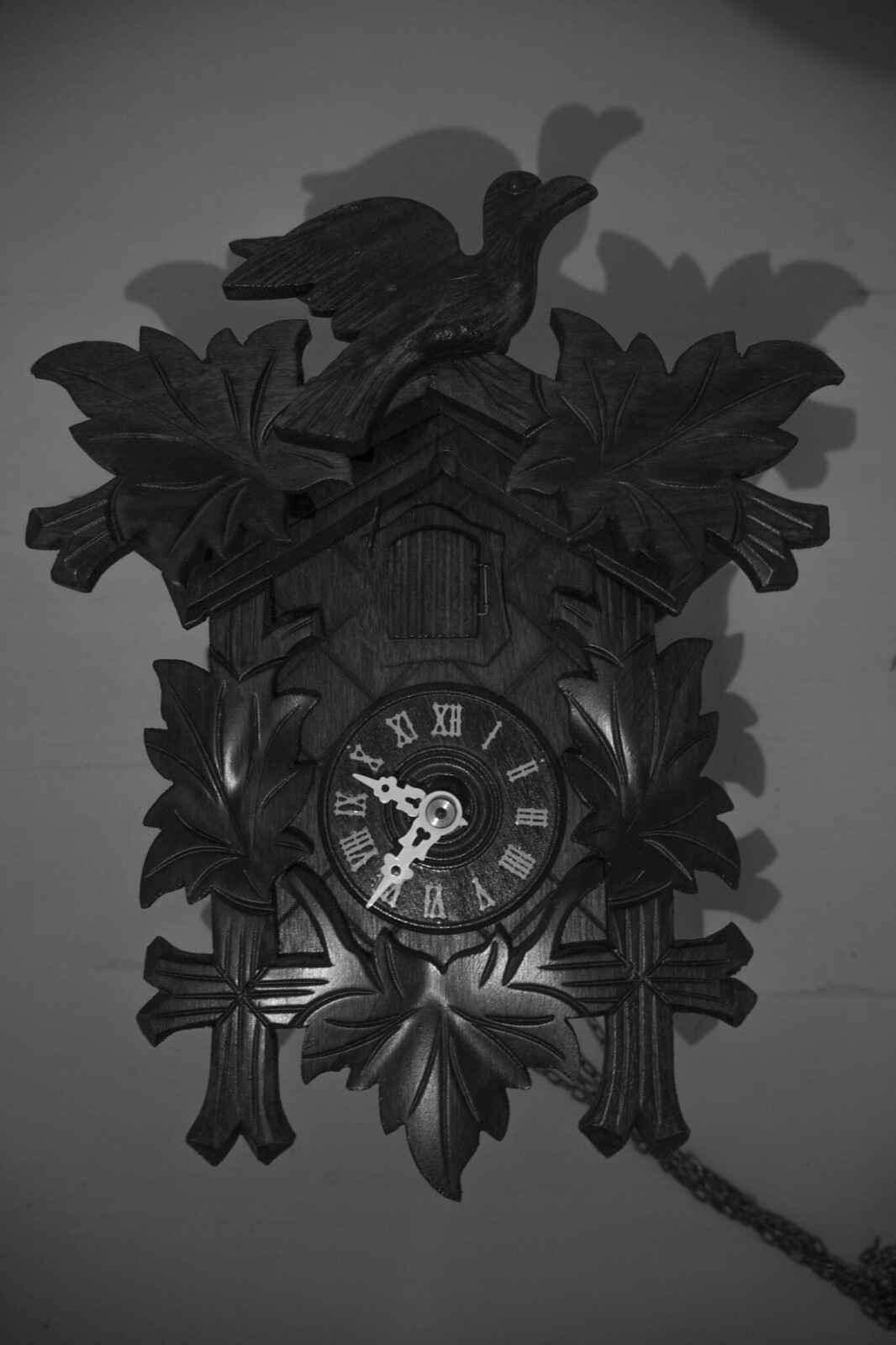This black and white photograph showcases an ornate and elaborately carved wooden cuckoo clock mounted on a grayish-colored wall. The clock is adorned with intricate details, featuring a bird carving, possibly a dove, perched at the apex and flanked by two leaves on either side. Surrounding the clock face are additional leaf and flower carvings, casting shadows on the wall that enhance the clock's decorative appeal.

The clock face displays white Roman numerals and light-colored hands, set to approximately 9:35. Above the face, a small wooden door, presumably for the cuckoo bird, remains closed. A chain hangs from the bottom of the clock, extending out of the frame's bottom right corner, suggesting a possible connection to an unseen object. The clock's intricate carvings, including cross-like details at the bottom corners and an additional leaf below the clock face, emphasize its vintage and elaborate design, indicative of a traditional cuckoo clock.